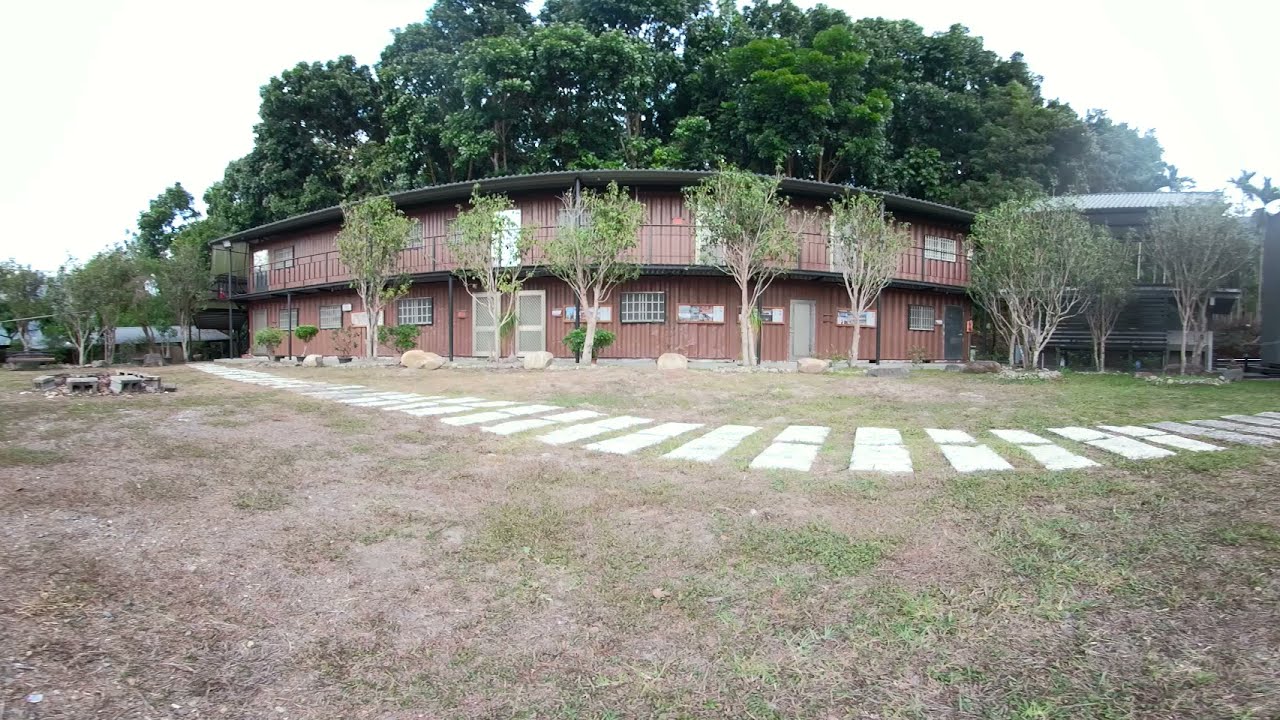This daytime outdoor photograph showcases a two-story rectangular building, likely a motel, with a distinctive curved exterior clad in vertical brown siding. The structure features multiple windows trimmed in black, spread evenly across both floors. The first level has several light brown doors and a gray door, while the second floor includes a few more doors, some of which are white, and a balcony or walkway connecting them. The roof is constructed of tin, adding a modern touch to the building's rustic appearance.

In the foreground, a sprawling lawn of greenish-brown grass, interspersed with patches of dead grass, stretches out before the building. A curved stone walkway, comprised of small rectangular white concrete blocks, meanders from the edge of the house, curving towards the center before veering to the right. This walkway is flanked by bare patches of grass and a makeshift fire pit bordered by cinder blocks on the left side. 

A row of five slender trees lines the front of the building, with much taller trees standing guard behind it, providing a dense backdrop. There’s also an impression of another structure with dark wood siding behind the trees on the right, partially obscured from view. Additionally, a taller green building is visible in the background to the right of the main structure. Overall, this image blends the charm of rural architecture with the serenity of nature.